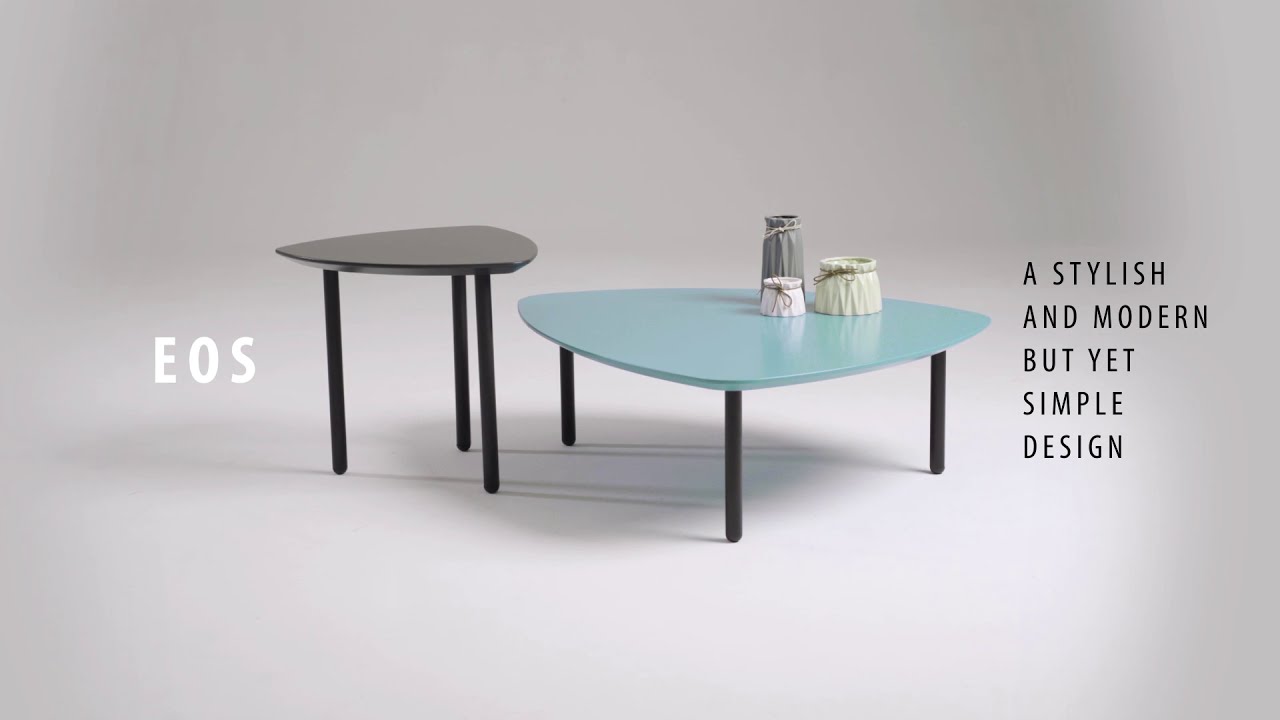The image features a minimalist indoor setting with a light gray background and subtle shadows. Central to the image, there are two triangular coffee tables. The larger central table is light blue with curved corners and edges, standing on three black legs—one leg positioned close to us and two aligned at the back. Atop this table, arranged meticulously, are three containers adorned with satchel bags: a small white one in front, a round, slightly grayish-white one to its right, and a tall slender gray container in the back. To the left of this central table, there is a smaller, taller black table with a similar triangular shape but devoid of any objects. 

The left side of the image prominently features the white letters "EOS," while the right side of the scene showcases black sans serif text that reads, "A stylish and modern but yet simple design," spread across five lines. The tables cast faint gray shadows onto the white floor, reinforcing the clean and elegant aesthetic. Overall, the arrangement and text suggest a sophisticated furniture advertisement.